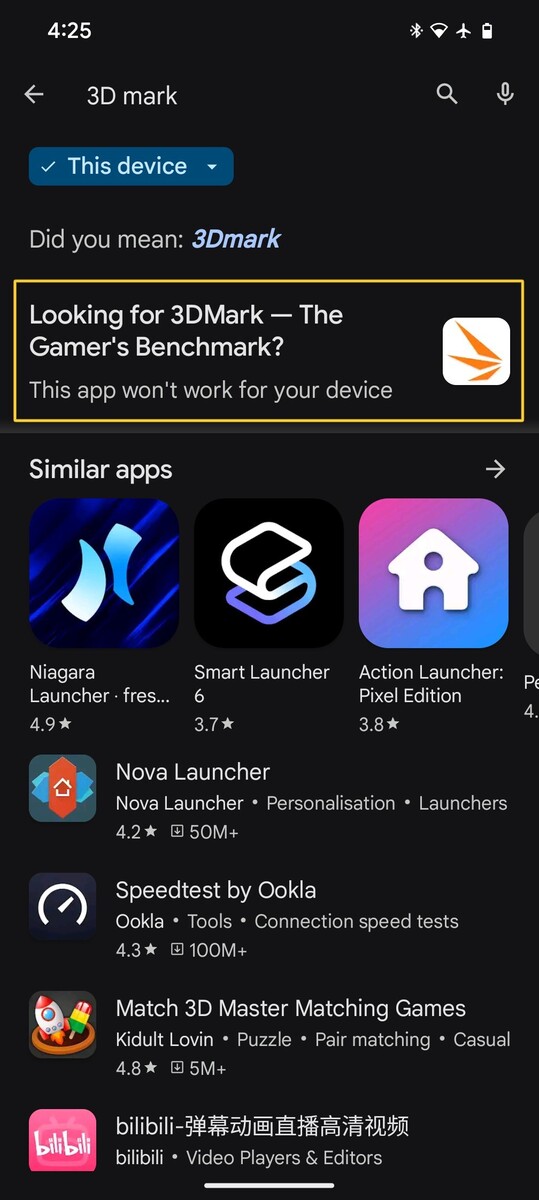This image is a screenshot from a smartphone using dark mode, characterized by a completely black background. 

In the upper left corner, the time is displayed as 4:25. On the upper right, a collection of white icons indicate the device's status: the battery is approximately two-thirds charged, and icons for airplane mode, Wi-Fi, and Bluetooth are also visible.

Below these status icons, there is a search box. To the left, "3D Mark" is written, accompanied by a white arrow pointing left, indicating a navigation option. On the right side of the search box are the search and microphone icons, signaling that this is likely a Google search feature.

Directly beneath "3D Mark," there is a blue rectangle resembling a drop-down menu, displaying options with a sky blue font. The text reads "This device," and beneath it is a suggested search correction: "Did you mean 3DMark?"—notably written as a single word. Following this, a question is posed: "Looking for 3DMark the gamers benchmark?" with a clarification that "This app won't work for your device."

Below this text, there are three app icons. The first, "Niagara Launcher," features a blue background with dark blue and royal blue diagonal stripes and sky blue crescent shapes. The middle icon, for "Smart Launcher," has a black background adorned with white and blue lines. The third icon, on the right, shows a partially sky blue, partially purple background with a white house in the center.

The overall scene suggests the user is browsing the Google Play website on their smartphone, searching for apps related to "3DMark."